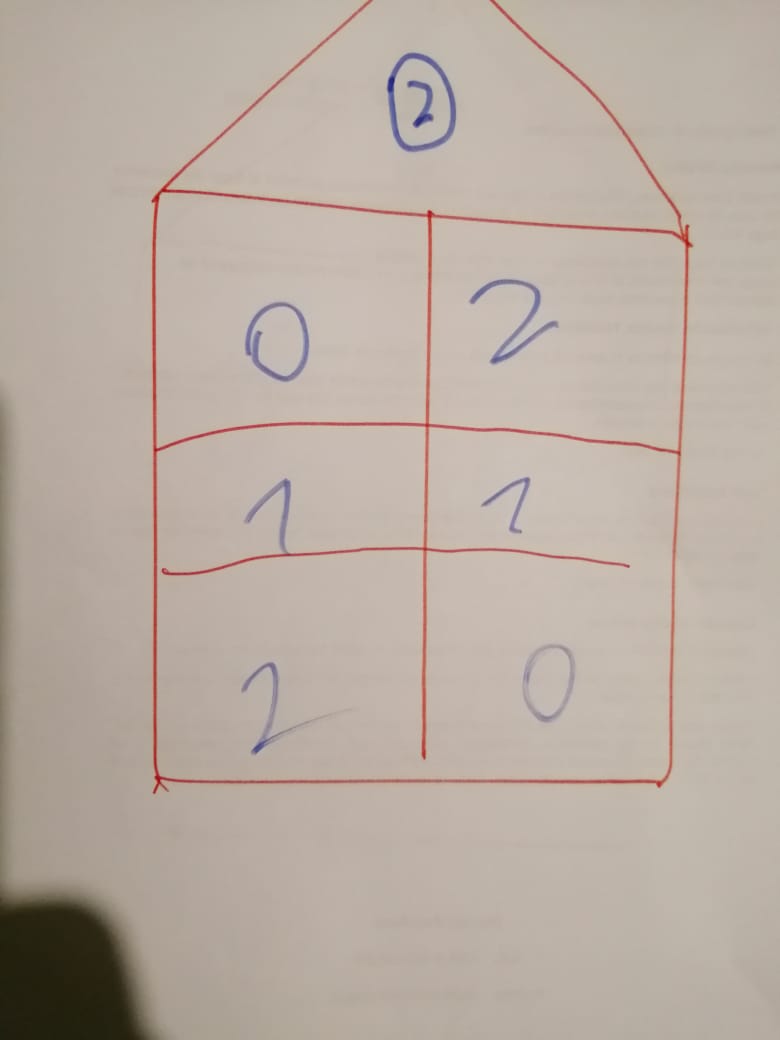The image displays a detailed sketch of a house structure outlined in red ink. The paper background is light gray, with a slight black shadow occupying the bottom left corner. The structure has a square base at the bottom, featuring two horizontal red lines; the bottom line does not extend to the right edge, while the top line does. A vertical red line in the center divides the square base, creating six smaller sections within it. Numerical annotations in faded blue ink are present: the bottom row reads "2" on the left and "0" on the right, the middle row reads "7," and the top row reads "0" on the left and "2" on the right. Above the square base, a triangular outline in red houses a blue circle with the number "2" in its center. This combination of geometric shapes and numbers constitutes the entire composition of the sketch.